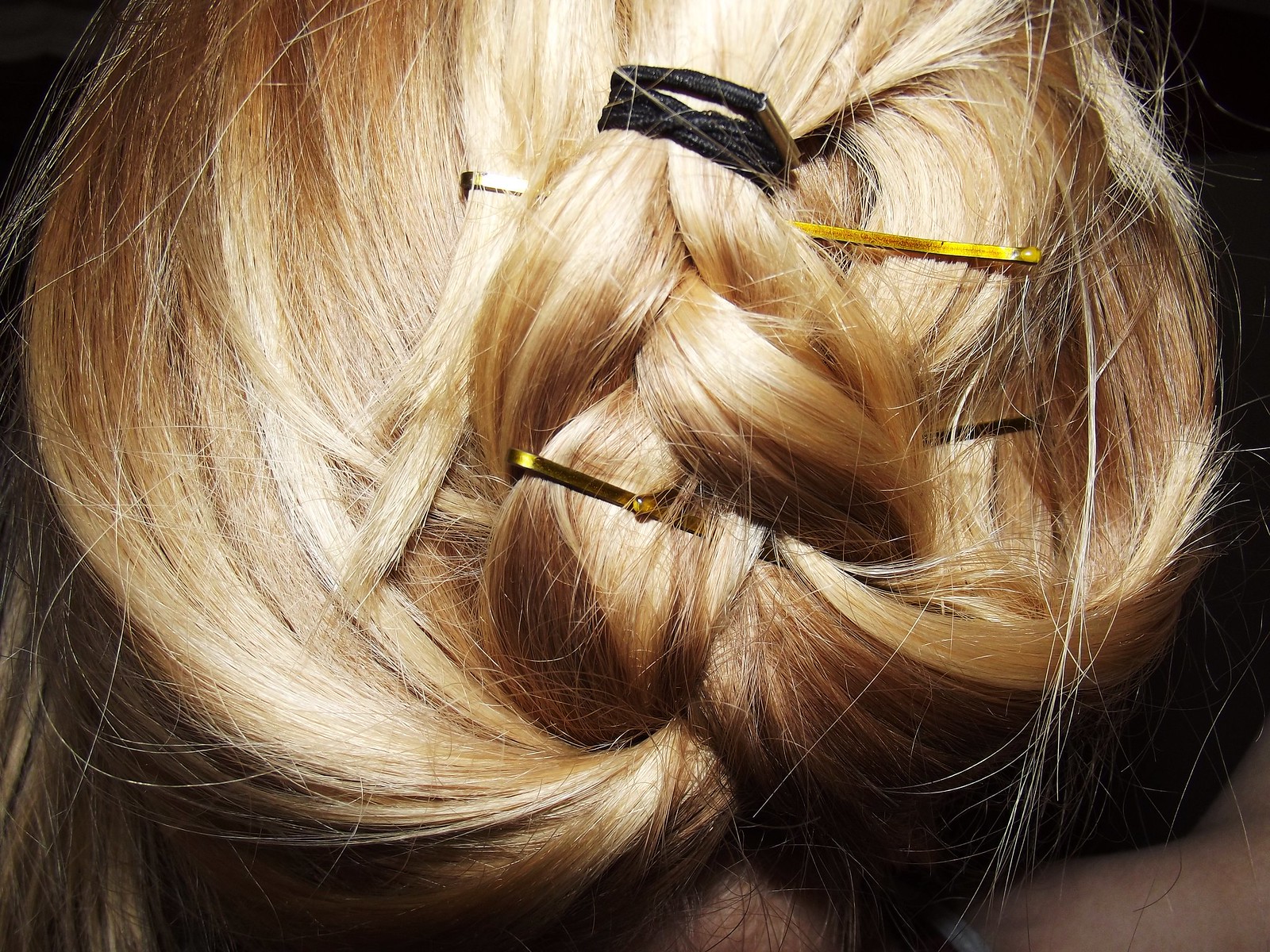The image showcases a close-up of the back of a woman's head, focusing on her intricately styled blonde hair. Her hair, featuring both pale blonde and darker blonde streaks, has been fashioned into a French braid secured at the top with a black elastic band. The braid is then artfully flipped upward and tucked behind itself, forming a bun. Strands of hair have escaped the braid, creating a soft, loose framing around her face, though not visible in this shot. The bun is held in place by approximately four yellowish-gold bobby pins, and the tail end of the braid can be seen peeking out from behind the bun. The image is tightly cropped, showing only a hint of her shoulder, with no view of her neck, face, or ears. The photograph emphasizes the intricate details of the hairstyle, highlighting the blend of loosely falling strands and the secure, pinned structure.